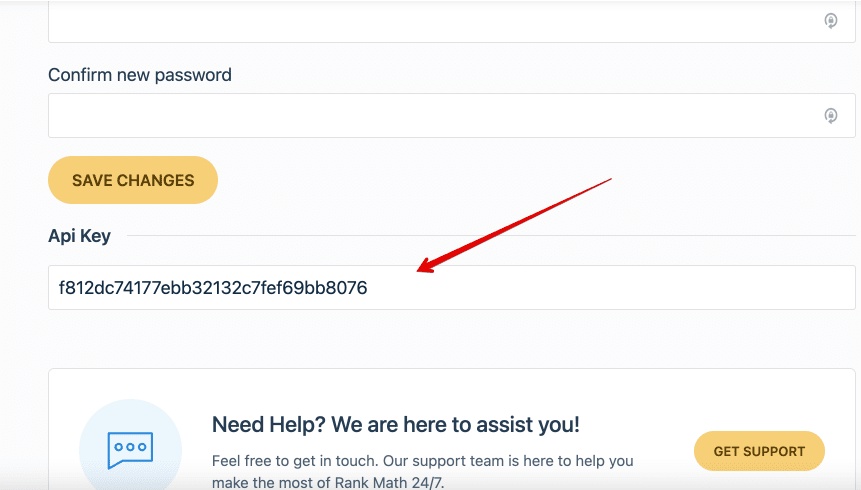The image captures a section of a website, showcasing a user interface primarily related to account settings and support. At the top, there's a white box with a red circular icon on the right side, possibly indicating an alert or notification. Below this, the text "Confirm New Password" is displayed, accompanied by an input box for the user to enter their new password. 

Further down, an orange button labeled "Save Changes" stands out against the interface. Below this button, the label "API Key" is prominently displayed in black text, followed by a white input box containing a lengthy alphanumeric string. A long red arrow points to this string, emphasizing its importance, akin to a confirmation code you might encounter in a Prolific survey.

Beneath the API key section, a gray box reads "Need Help? We are here to assist you." Next to this is a light gray circle containing a conversation icon with three dots, symbolizing an active chat or support option. The accompanying text encourages users to contact support: "Feel free to get in touch. Our support team is here to help you make the most of Rank Math 24/7." To the right of this text, another burnt orange button with smooth edges is labeled "Get Support," inviting users to seek assistance whenever necessary.